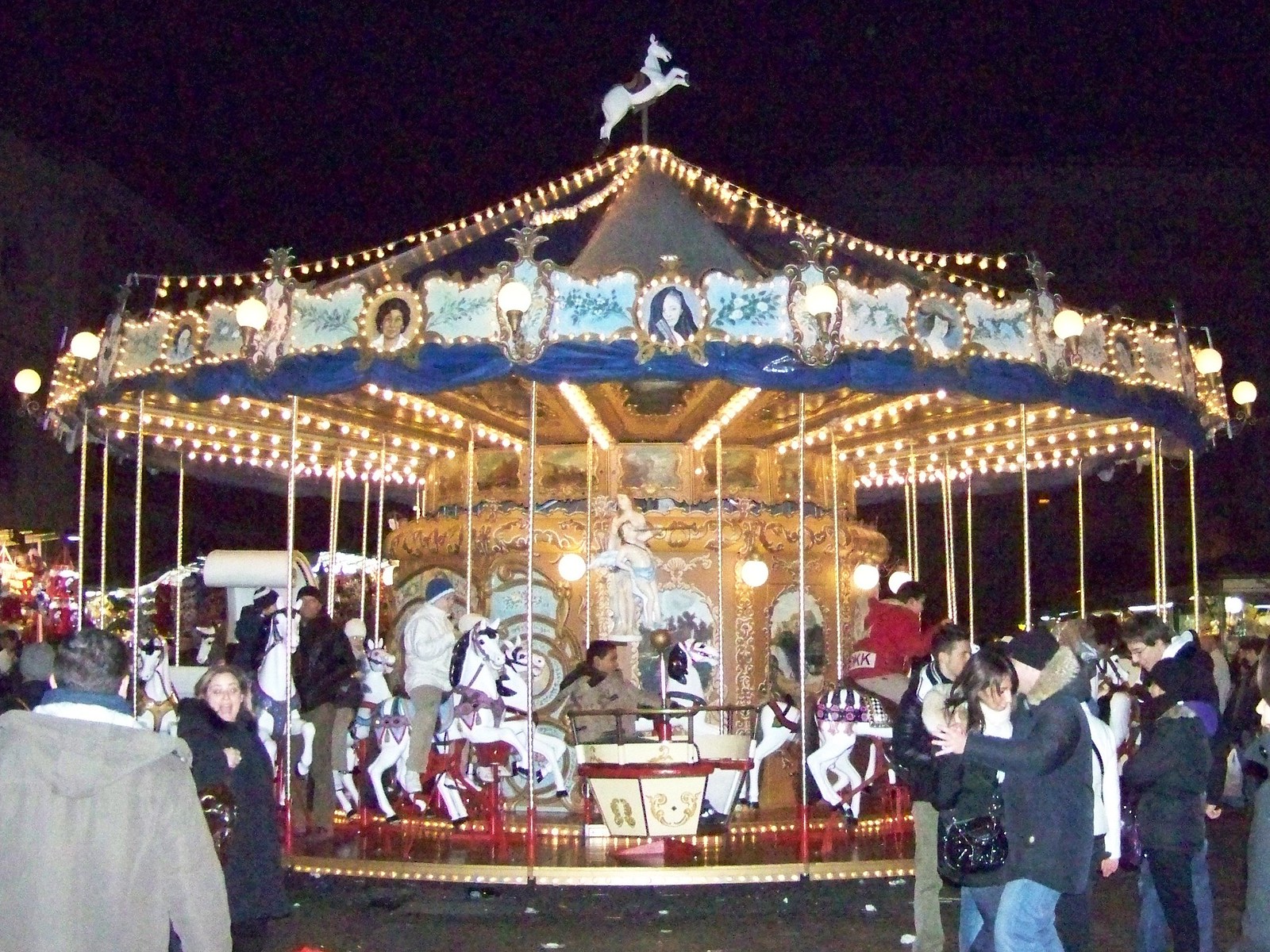The photograph captures a lively night scene at an amusement park or county fair, centered around a beautifully lit carousel. The carousel, adorned with regal gold accents, mirrors, and a string of bright yellowish lights, features traditional white carousel horses with blue and purple trappings, as well as stationary seats and a small wagon for riders. The scene is bustling with people, some of whom are riding the carousel while others stand around observing or waiting to board. Many of the individuals are dressed in heavier jackets, suggesting a chilly evening. In the background, food stands add to the festive atmosphere. The merry-go-round is packed, and the entire area exudes a joyful energy, making it a focal point of celebration and amusement amidst the dark night sky.